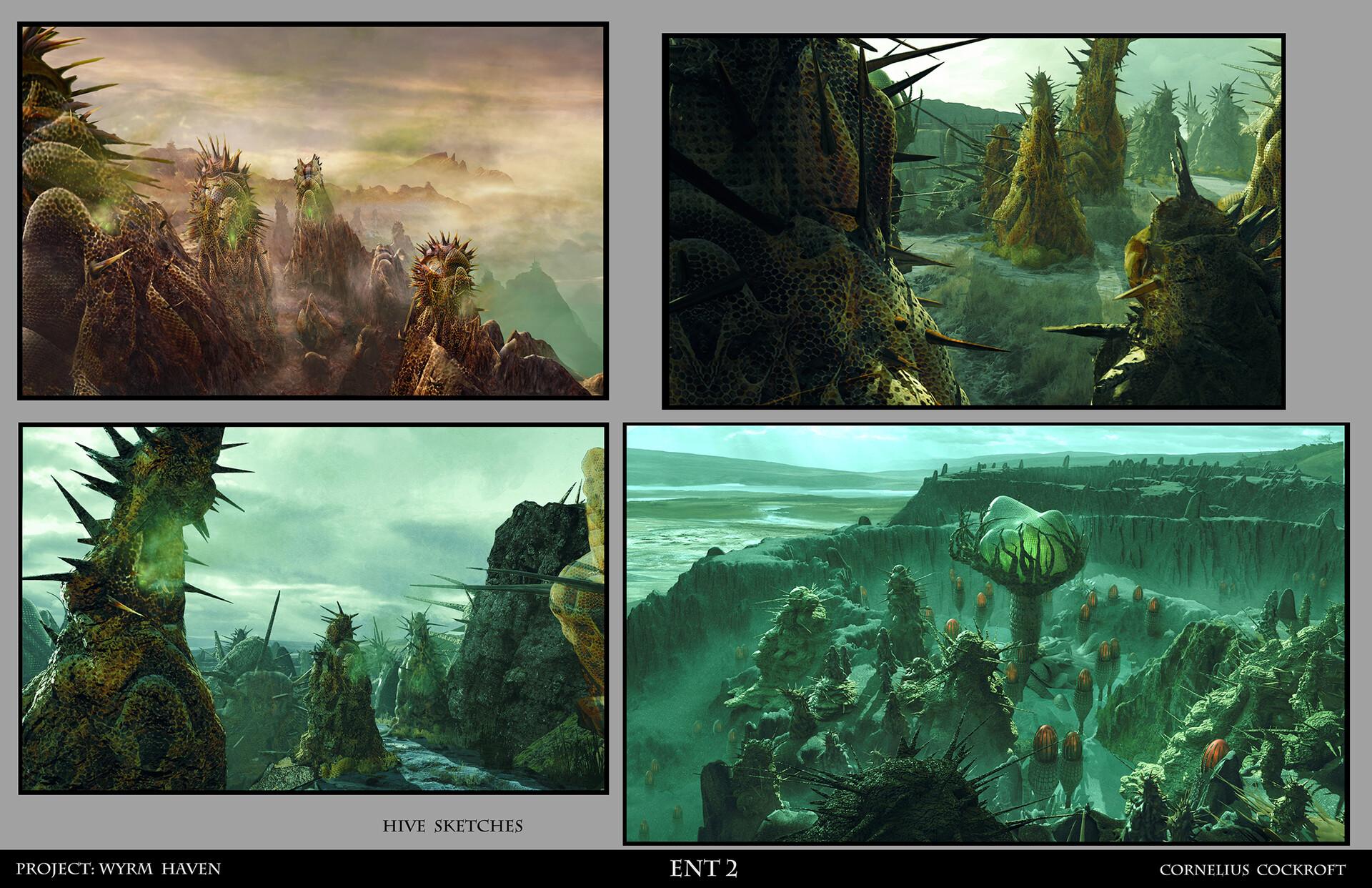The image is a composite of four distinct panels, all set against a gray background, and appears to be part of a storyboard or concept art for a fantasy or sci-fi setting, possibly for a game or a website. The top left panel showcases rugged mountains enveloped in clouds or plumes of smoke, creating a mystic atmosphere. Adjacent to it, in the top right panel, vibrant green, thorny plants stand out, their intricate details vivid against the gray backdrop. The bottom left panel features blue-tinted rocky formations, adorned with thorn-like protrusions, which conjure a surreal, otherworldly landscape. The bottom right panel presents a rocky mountainside dominated by a towering, cactus-like structure brandishing a glowing green orb or goblet at its center, surrounded by smaller glowing bulbs and spiky columns. The entire composition is labeled "Hive Sketches" and features a black annotation at the bottom that reads "Project WYRM Haven ENT 2 Cornelius Crockcroft."